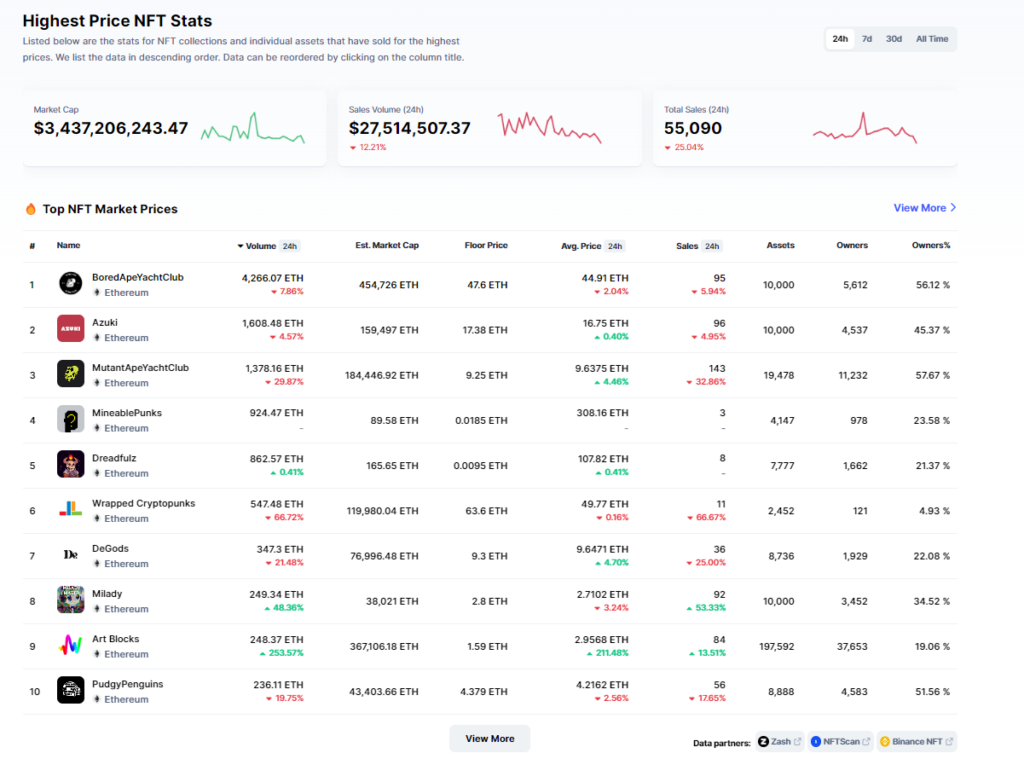This screenshot displays detailed NFT information on a website, set against a light gray background that lightly gradients to white at the bottom. At the top left corner, "Highest Price NFT Stats" is written in bold black text. Below this title, a paragraph in light gray text provides an explanation: "Listed below are the stats for NFT collections and individual assets that have sold for the highest prices. We list the data in descending order. Data can be reordered by clicking on the column title."

In the top right corner, within a medium gray box, there are four filter options. The first option, "24 hours," is highlighted in white, while the other options, "7 days," "30 days," and "All time" are presented in gray.

The section below displays three information boxes with white backgrounds and rounded corners. The leftmost box shows "Market Cap" with an amount of $3,437,206,243.47, accompanied by a green line chart on the right. The center box provides "Sales Volume (24 hours)" amounting to $27,514,507.37, with red text beneath that indicates a decline of 12.21% and an arrow pointing down next to a red line chart. The rightmost box shows "Total Sales (24 hours)" which is $55,090, also down by 25.04% as indicated by red text and an arrow pointing down, accompanied by another red line chart.

Below these boxes, there are rows of detailed information under the heading "Top NFT Market Prices." The listed columns include "Name," "Volume (24 hours)," "Estimated Market Cap," "Floor Price," "Average Price (24 hours)," "Sales (24 hours)," "Assets," "Owners," and "Owners Percent." The data for the corresponding rows is listed beneath these columns, providing a comprehensive view of the NFT market prices.